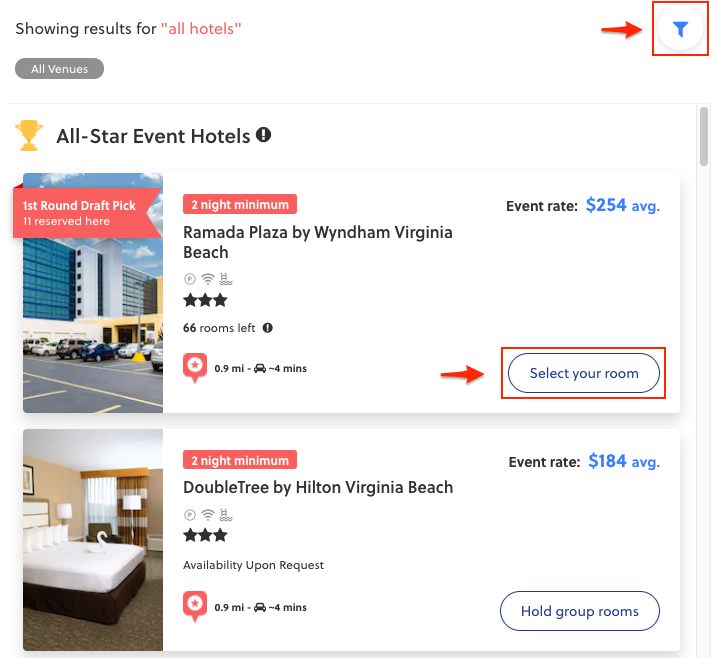The image is a screenshot from a hotel booking website. In the upper left corner, the text "Showing results for 'All Hotels'" is displayed, with "All Hotels" highlighted in red quotation marks. Below this header, a small yellow trophy icon appears next to the phrase "All Star Event Hotels."

The screenshot features two hotel listings, each presented in rectangular boxes spanning horizontally across the screen against a mostly white background with black text. Each listing includes a small image on the left side.

The first listing showcases the exterior of a hotel, a modern building with blue and gray accents. The text details the hotel as "Ramada Plaza by Wyndham, Virginia Beach," rated three stars, with "66 rooms left." An eye-catching red arrow points at a box in the lower right corner that says "Select your room," which is also circled in a red rectangle.

The second listing features a photograph of a hotel's interior, specifically a room decorated with white and brown bedding, a tan accent wall, matching brown and tan curtains, and brownish carpeting. This hotel is identified as "Doubletree by Hilton, Virginia Beach," also rated three stars, with "Availability upon request" noted. The event rate is listed at an average of "$184." In the bottom right corner, a blue oval button labeled "Hold Group Rooms" is prominently displayed.